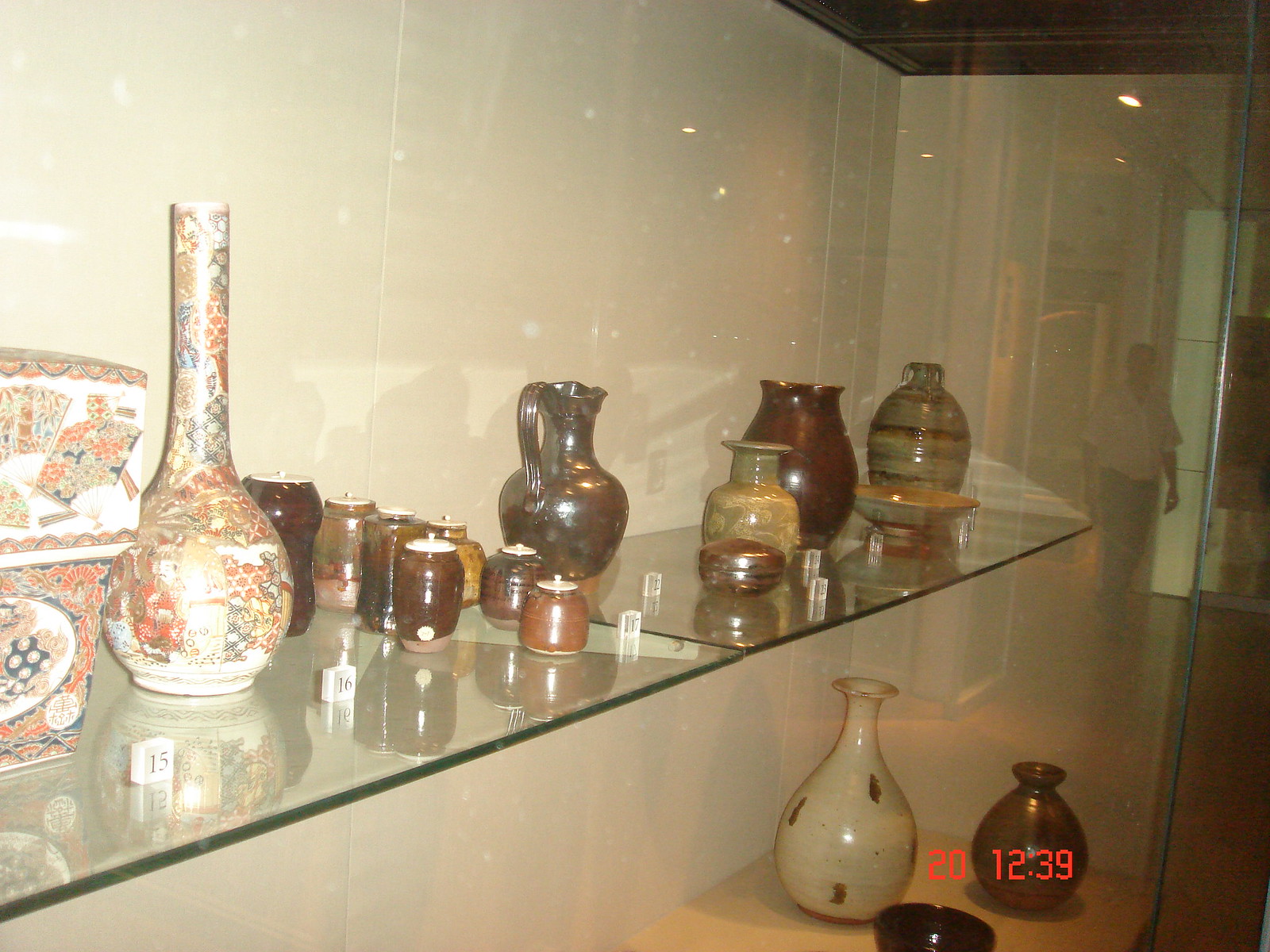This photograph captures a large glass display case situated against a wall, reminiscent of an exhibit at a museum, auction, or specialty resale shop. The case features a front and sides made of glass, and inside, there is a glass shelf that holds an intricate collection of glassware, including pitchers, urns, vases, and other small containers, many with lids. Each piece is paired with a small white block displaying a black number, suggesting that they are sets or lots available for sale or auction.

The objects inside the case are diverse in design and color. Notably, on the left side, there are two vessels adorned in an Asian style, showcasing a palette of red, dark blue, gold, white, and brown. Adjacent to these are smaller vessels painted in variegated shades of brown, dark green, and gold. Among the collection, a dark gray pitcher with a single handle stands out, along with urns in colors ranging from jade green to bronze. One urn features stripes of jade green, brown, and yellow.

A shallow gray bowl is also part of the display, while on the bottom shelf, a tall vessel stands wide at the bottom with a narrow neck, its white surface speckled with darker spots. Another vessel with a similar shape but shorter and brown in color complements it. The glass reflection reveals a man dressed in a white button-up shirt and dark trousers, adding a subtle human element to the scene. An older date and time watermark, reminiscent of old camcorder recordings, is also visible on the image, adding to its vintage feel.